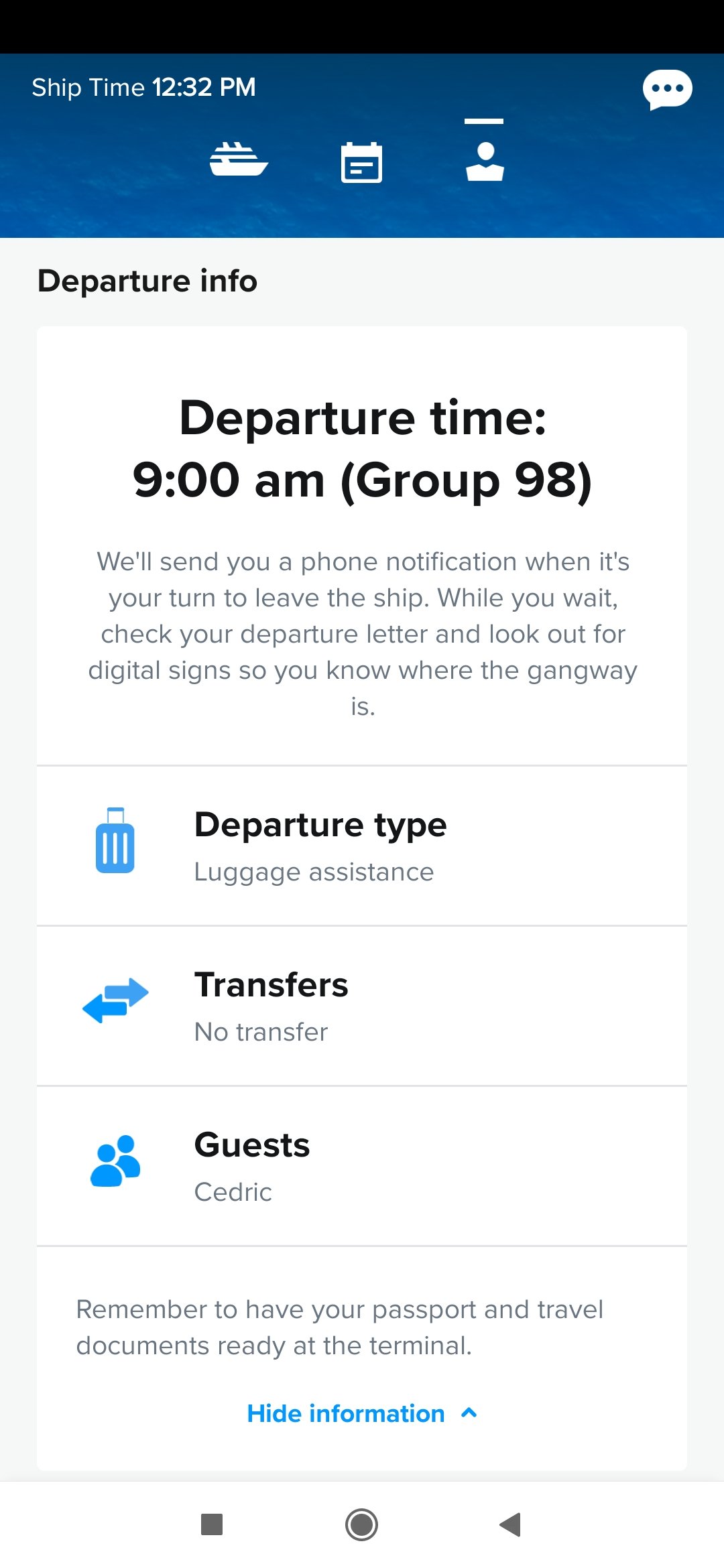This image displays a phone notification regarding the departure details for a boat. At the top of the screen, there is an icon of a boat, indicating that the notification concerns a ship departure. The main text reads "Departure Info" and specifies the departure time as 9 a.m. for group 98. It also mentions that a phone notification will be sent when it is time to disembark the ship. The notification advises passengers to check their departure letter and look for digital signs to locate the gangway.

Further details include:
- **Departure Type:** Luggage Assistance
- **Transfers:** No Transfer
- **Guests:** Cedric

A reminder at the bottom asks passengers to have their passport and travel documents ready at the terminal. There is also an option to "Hide Information," likely allowing users to minimize the notification on their phone. The text is primarily in black on a white background, with a blue ribbon at the top containing various icons, and some light blue icons interspersed within the white area containing the black text.